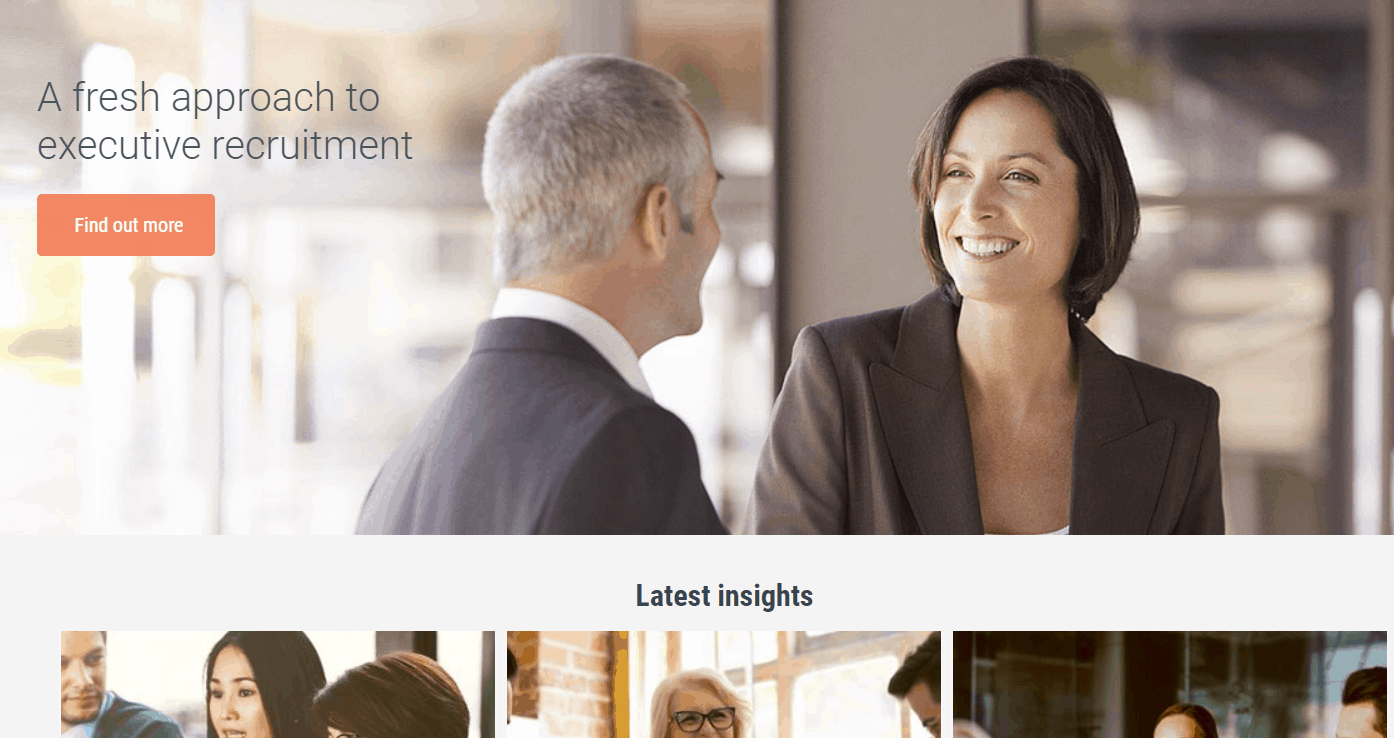This executive recruitment website features a prominent tagline at the top that reads "A Fresh Approach to Executive Recruitment" in bold black letters. Just below this tagline is a call-to-action button with the phrase "Find Out More" in white letters, encased in a red border and background. 

The site's background boasts a collage of four images, each depicting various business meetings. The largest image, positioned next to the headline, showcases a man and a woman engaging in a professional discussion. They appear to be in a modern office or a casual coffee shop setting. The woman, who is smiling, is dressed in a brown suit blazer over a white top and has short, dark brown hair. The man, seated opposite her, is wearing a black suit with a white shirt, and although his face isn't visible, his short gray hair is noticeable.

Below this main image, three smaller pictures illustrate different business meeting scenarios. The first shows two women in conversation, with a man attentively listening to them. In the second image, a woman wearing glasses is speaking while two men focus on her. The third image captures just the tops of the heads of three individuals: two men with brown hair and a third person with blonde hair.